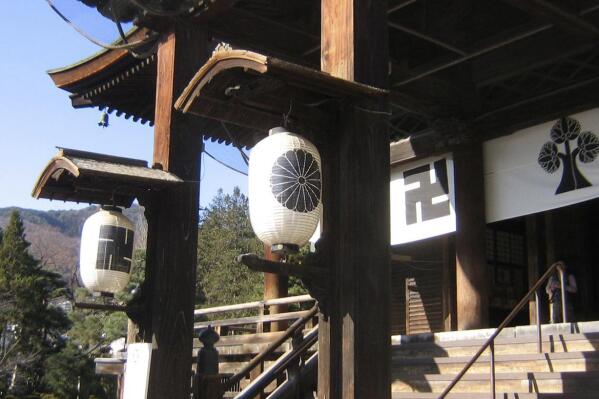This image captures a detailed close-up of the entrance to a traditional Japanese Buddhist temple. The temple, constructed from medium brown wood, features iconic curved eaves and intricate wooden decorations. The stairs leading up to the entrance combine old-fashioned wooden railings with modern metal supports. Hanging above the entrance are two oval paper lanterns, one adorned with a black mandala-like design and the other with a non-tilted Buddhist swastika, both symbolic in Buddhist culture. White banners featuring tree designs and additional black swastikas run around the building. The backdrop showcases lush pine trees, a forested mountain, and a clear blue sky, adding to the serene and picturesque setting of the temple.